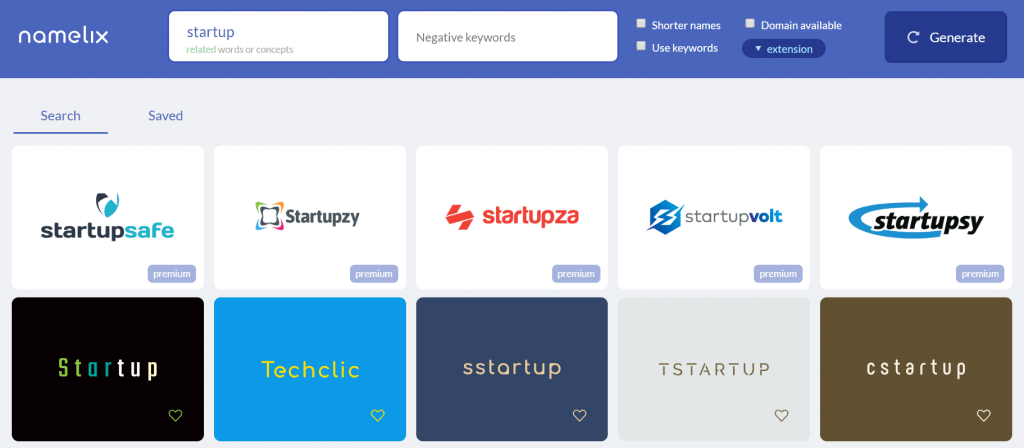This image showcases the NameLix website, prominently featuring a blue header at the top. The website interface includes two white input bars: one labeled "Startup" for related words or concepts, and the other designated for "Negative Keywords."

In the blue header box, there are options such as "Shorter names," "Use key search," "Domain available," and "Extension." A "Generate" button is located in the right corner of this section. Directly below, a gray navigation bar contains the words "Search," underlined in blue, and "Saved," also highlighted in blue.

The image further displays a series of individual name suggestion boxes, each varying in color. The first box, white, shows "Startup Safe," with "Startup" in black and "Safe" in green. The next box presents "Startupsy" in green, followed by "Startupza" in red. The fourth box reads "Startup Vault," with "Vault" in blue and "Startup" in black. The fifth highlighted box, “Startupsy,” features a blue arrow looping around it.

Below this, an additional row of name suggestions includes: "Startup" in black, "Technic" in blue, "ssStartup" in navy, "tStartup" in beige, and "cStartup" in brown.